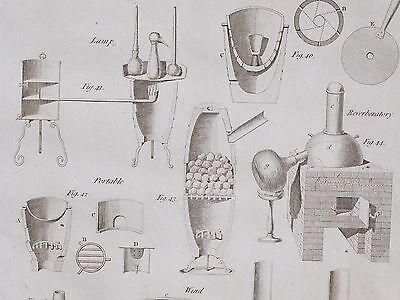This black and white illustration, reminiscent of patent drawings or an old encyclopedia, meticulously details various components and cross-sectional views of what appears to be a sophisticated heating or distillation mechanism. The diagram consists of approximately ten individual drawings, some of which are cutaway images revealing internal structures. The central focus seems to be on a brick-like apparatus with an open metal door, a hemispherical top, and a smokestack-like tube protruding from it. Additional images show intricate internal parts arranged inside a large drum-like structure, suggesting a kiln or a still for laboratory use. The illustrations are finely detailed, employing shades of black, white, and gray, with accompanying cursive text that is difficult to decipher. This comprehensive diagram provides an in-depth visual breakdown of the device, capturing its various elements, many of which appear designed to handle heat or facilitate the distillation process.